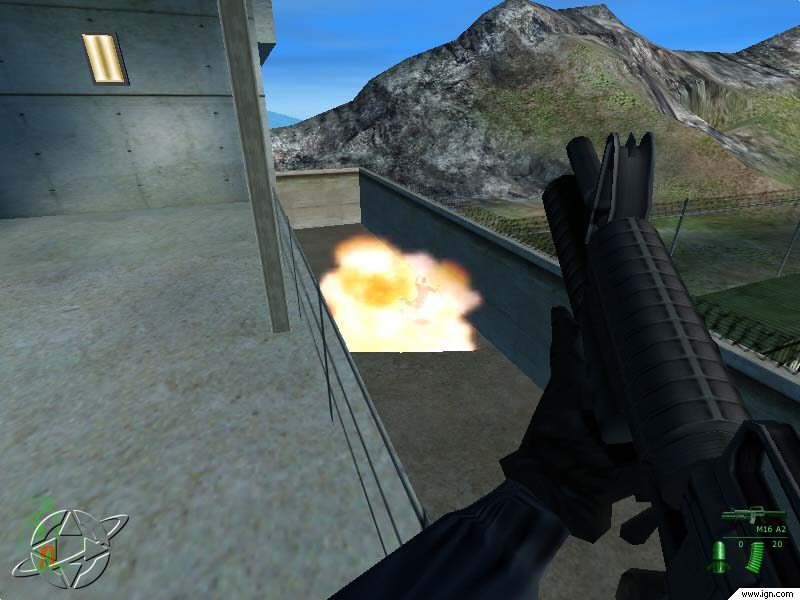The image is a detailed color screenshot from a live play session of an old-style computer game reminiscent of the early Wolfenstein days but with more advanced 3D graphics. In the bottom right foreground, the player's character is depicted, identifiable by a silhouetted black-gloved hand gripping a black machine-style gun, similar to an AK-47. The gun is tipped upwards at a 45-degree angle, suggesting recent discharge. The middle of the screen is dominated by a fiery explosion, vividly rendered with a central yellow hue and darker orange detailing at the edges. In the midst of the explosion, the faint outline of a body is visible, with a head, arms bent at the elbows pointing upwards, torso, and legs flung outward, indicating a direct hit by a rocket-propelled grenade. The scene is set on a rooftop with a gray guardrail, overlooking a backdrop of blue sky and a mountainous area that features greenery and possibly a stream. A meter display and directional arrows in the lower right corner provide the player with vital game information, such as remaining ammunition. The building appears to be constructed from concrete or metal, suggesting a fortified patrol position under attack.